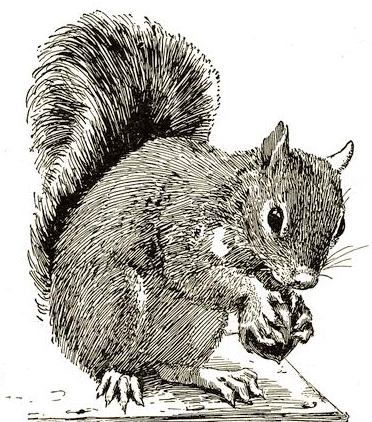This is a detailed pencil and pen sketch of a squirrel, depicted in black and white, standing on a wooden board or platform, set against a white background. The squirrel is facing slightly to the side with its head bent down, as if about to eat a nut it holds in its tiny hands. Its eyes are open and almond-shaped, and its ears are perked up, adding to its alert expression. Notably, the drawing captures the intricacies of the squirrel's anatomy with visible toes and toenails, as well as the bushy tail that stands erect behind it, making it the tallest part of the squirrel. Delicate whiskers extend from its nose, which is small and olive-shaped. The sketch is quite detailed, highlighting the texture of the squirrel's fur, with some darker sections, especially on the tail. This charming and meticulous rendering emphasizes the squirrel's lifelike and cute appearance.